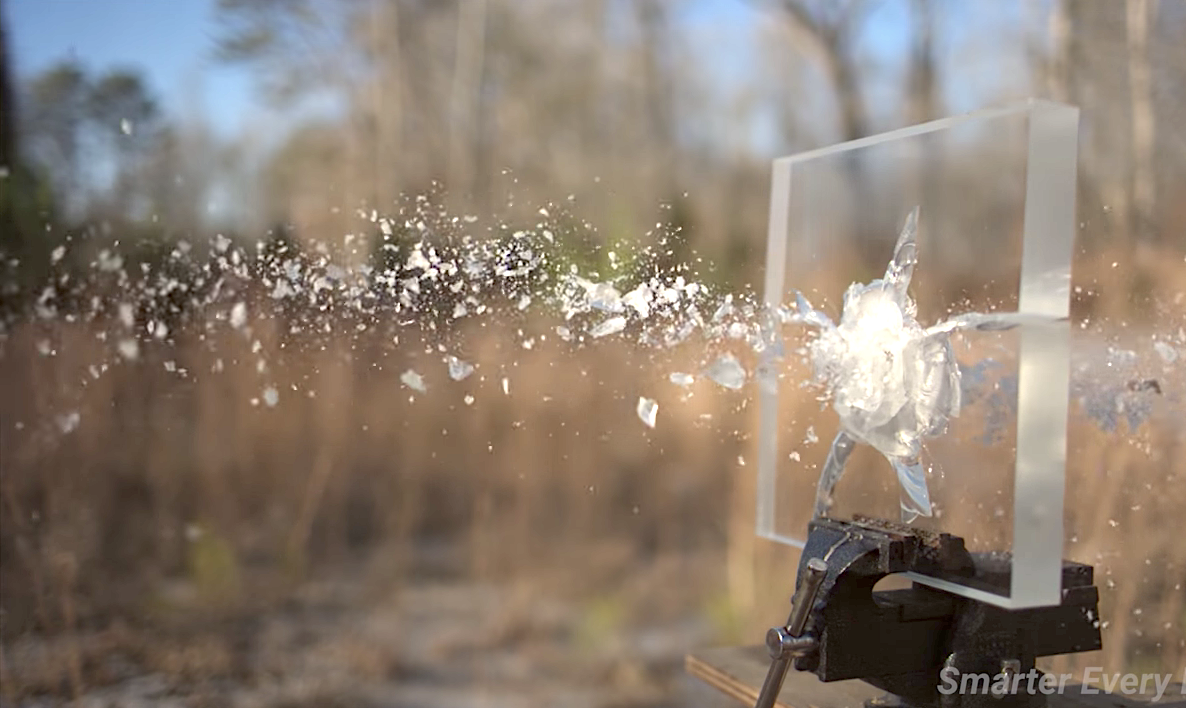In this dynamic color photograph, we see a thick, translucent glass panel, approximately two inches thick, held upright by a black metal workshop vise. The glass is in the midst of being shattered by a bullet, which has just punctured through its surface, creating a dramatic display of cracks and flying glass fragments. The shattering impact originates from the bullet hole near the center, splitting the panel horizontally and scattering particles in mid-air, capturing a vivid moment of destruction. The background reveals a tranquil outdoor setting with tall, green and rust-colored trees slightly blurred, and a clear blue sky above. In the lower right corner of the image, the text "Smarter Every" is visible, implying an educational or informative context for the picture. The metal fixture firmly grips the glass, highlighting the intentional and controlled nature of the shot.